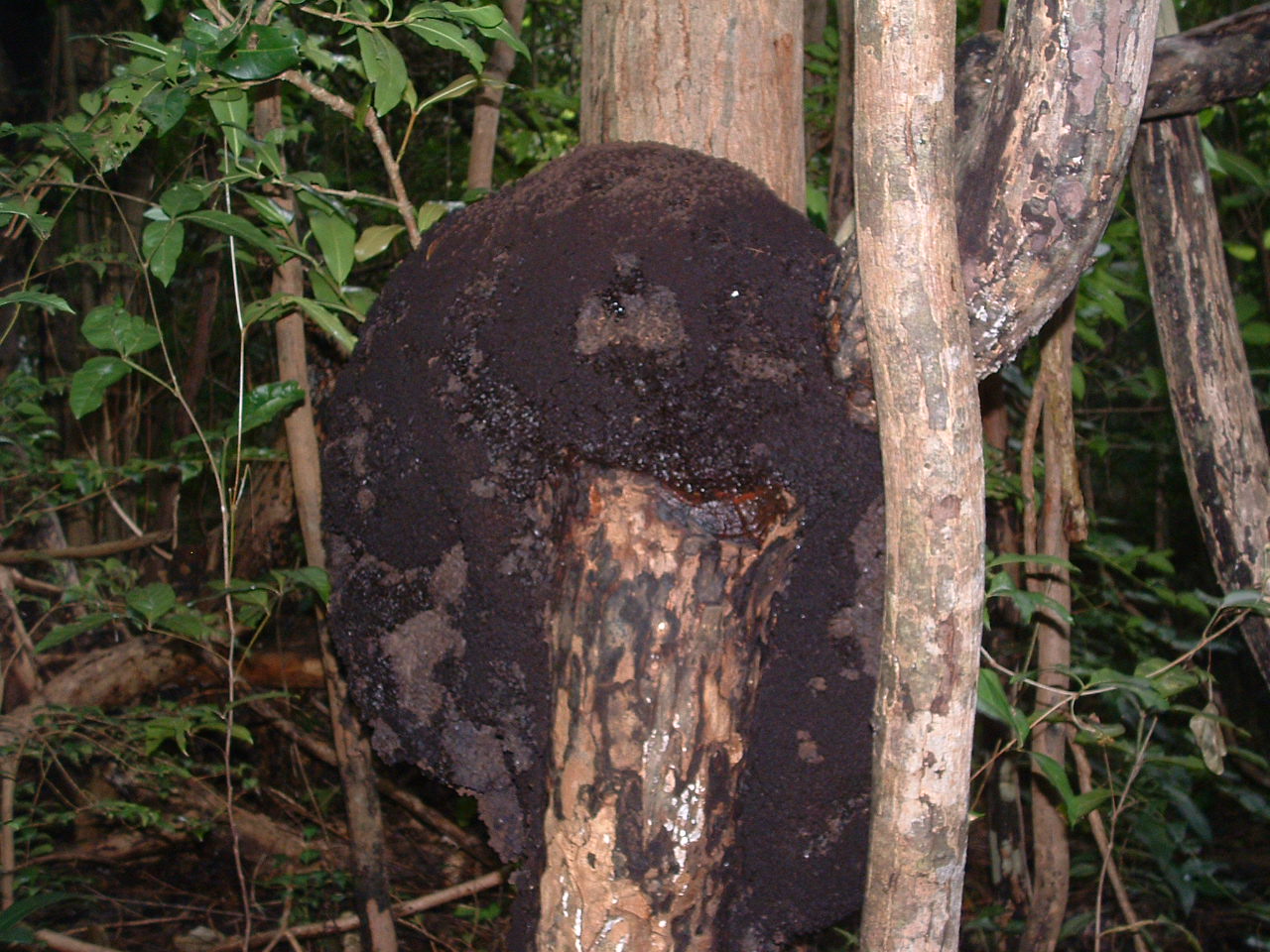This image features an outdoor forest or jungle scene, vividly capturing a densely vegetated area. In the left half of the picture, the background shows a wooded area with twigs scattered on the ground. Upper left reveals some green-leafed weeds or plants. Dominating the center is a large tree trunk, adorned with a mysterious black, mossy or possibly insect-like growth enveloping its top portion, creating an almost arm-like extension downward. The trunk itself is brown with contrasting black and light brown patches. To the right of this centerpiece, another thinner tree trunk rises, and in the far right corner, more twigs and smaller branches with green leaves are visible. The harmonious mix of nature's elements presents a captivating view of forest life, saturated with chocolatey dark hues, light tan bark, and lush green foliage.